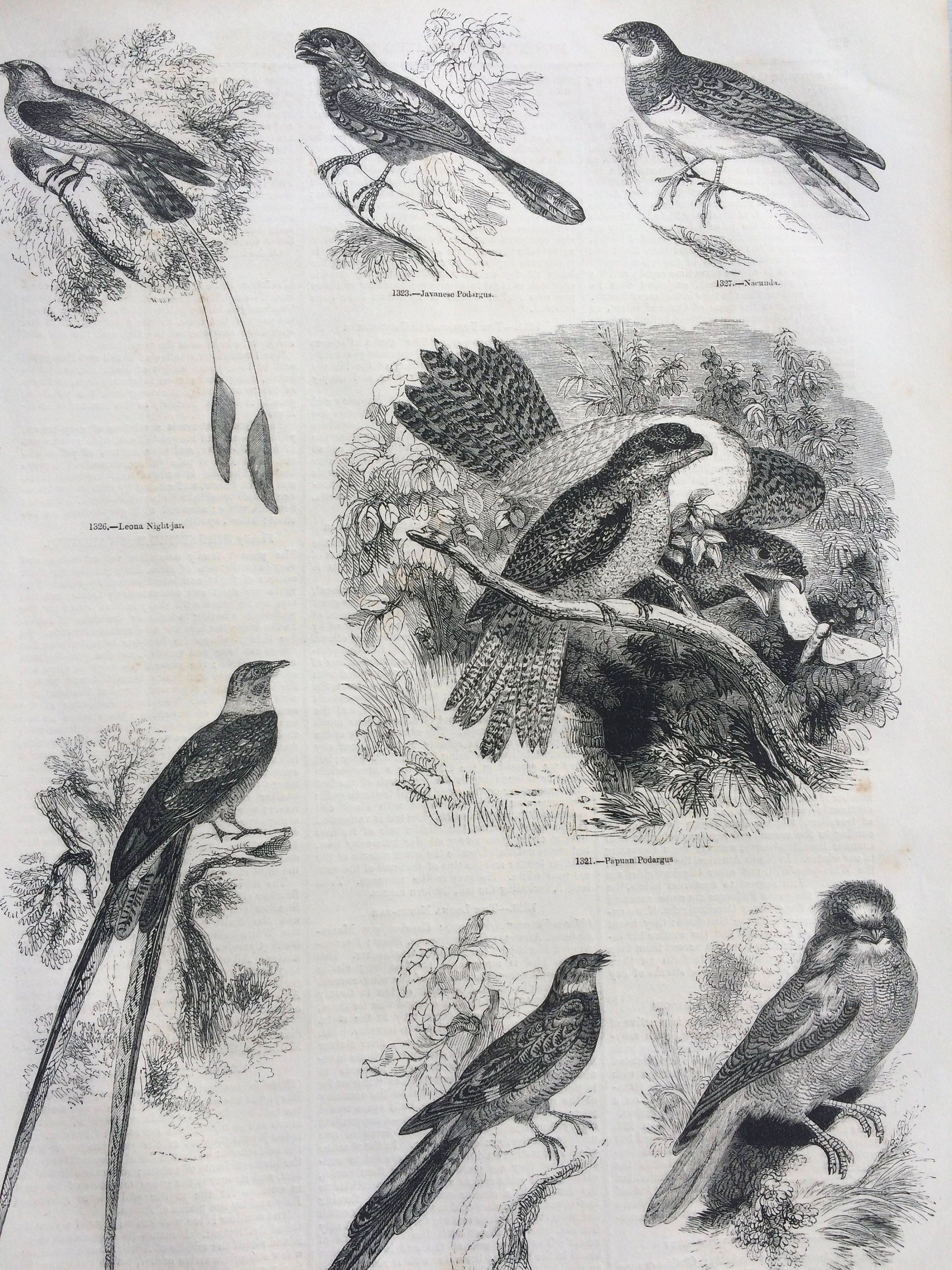This detailed drawing, created with black pencil on white paper and set against a light gray background, measures approximately 6 inches high by 4 inches wide and features multiple birds in various arrangements and poses. At the top, there are three distinct birds perched on a single branch, all facing left. These birds include a Leona Nightjar (1326), a Havanese Podargus (1323), and what appears to be a Nacunda (1327). In the center-right of the image, two birds, identified as Papuan Podargus (1321), are shown on another branch, with one appearing poised to eat an insect. The bottom section of the drawing features another trio of birds, all oriented to the right with one having a notably long tail, although their names are obscured. The artwork is highly detailed, with precise lines and a focus on the birds' unique characteristics, making it a beautifully intricate pencil drawing.